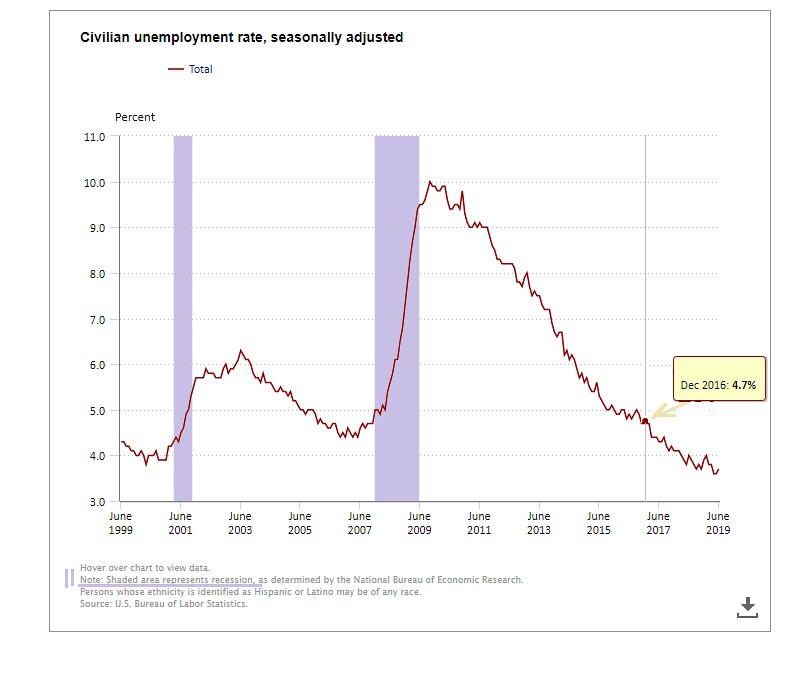The image is a detailed, seasonally adjusted graph titled "Civilian Unemployment Rate," with data spanning from June 1999 to June 2019. The graph is encased in a gray border on a white background, and prominently features a red line annotated as "total" in a key. The vertical axis, labeled with percentages from 3.0% to 11.0%, marks the unemployment rates, while the horizontal axis lists dates from June 1999 to June 2019. Notable peaks in the unemployment rate occur around June 2003 and June 2009, with the latter peak just after a thickly shaded blue area indicating a period of high unemployment between June 2007 and 2009. Another significant, albeit thinner, blue highlight spans June 2001 to June 2009. A yellow box with an arrow points to December 2016, marking a rate of 4.7%. The line graph typically fluctuates, with the highest value around 10.0% occurring close to 2010. Additional minor rifts can be seen throughout the timeline.